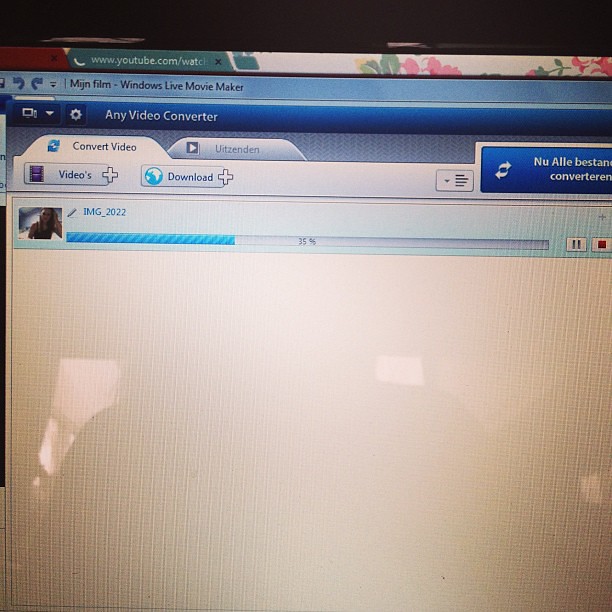The image captures a computer screen, possibly from a home or work setting, showing several windows and applications open. At the very top, there is a web browser tab displaying www.youtube.com. Below this tab, the active window is "MIGN Film - Windows Live Movie Maker." Next in line is an application with the title "Any Video Converter." 

Within this application, a specific task is highlighted: a video is being converted. The screen displays a snippet of a video featuring a blonde woman labeled "IMG_2022," and there is a progress bar indicating the download status which is at 35%, with a blue line progressing over a gray bar. Additional tabs include options labeled "Convert Video" and another that reads "Uitzenden," which is not currently selected. The screen is white underneath the progress bar, and there are reflections hinting at the light conditions in the environment.